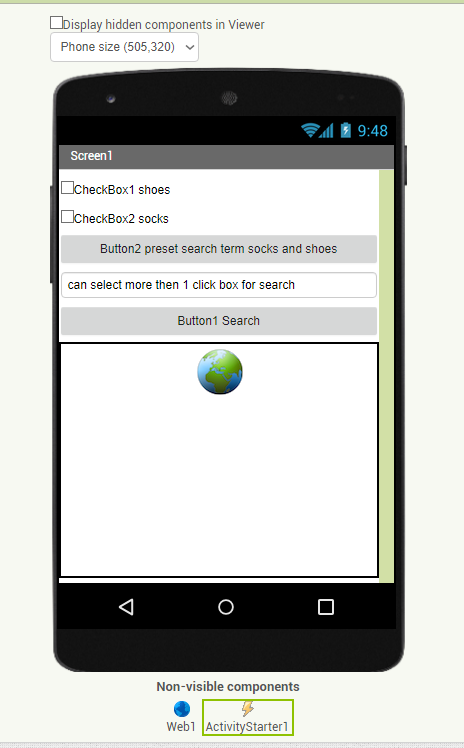The image depicts an unusually shaped and stretched-out device, which could either be a small phone or a pager, shown in a horizontal orientation. The device features a predominantly black frame with a white screen displaying a complex interface.

At the top of the screen, text reads "Display Hidden Components in Viewer" in gray, followed by what appears to be dimensions or a reference number: "(505,320)". Below this, the interface presents an image of planet Earth, with green representing the landmasses and blue the oceans. Flanking the globe is a light green sidebar.

Further down, the screen displays a header, "Screen One", with a series of interactive elements underneath:
1. An empty checkbox labeled "Checkbox One: Shoes".
2. Another empty checkbox labeled "Checkbox Two: Socks".

Adjacent to these checkboxes, gray text indicates the presence of a button labeled "Button Two: Preset Search, Term: Socks and Shoes". A note in white text underneath states, "Can select more than one, click box for search."

Towards the bottom of the screen, additional text in gray reads "Button One: for Search," following the note about the preset search button. Below the globe and these elements, the screen remains largely white, with a footer listing non-viable components: "Web One" and "Activity Starter One".